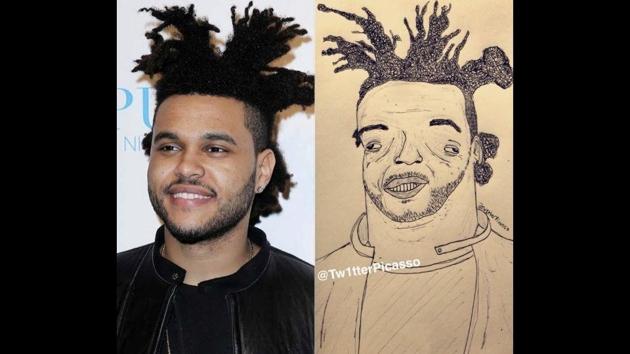The image consists of two side-by-side representations of the same individual. On the left is a photograph of The Weeknd, featuring his distinctive hairstyle with dreadlocks styled into various tendrils emanating from the top, akin to an upside-down mop or coral reef. He is smiling, showcasing his white teeth, and is dressed in a black shirt paired with a black leather jacket. His face is adorned with bushy eyebrows and minimal beard shading. To the right is a humorous and poorly executed caricature of him by Twitter Picasso, illustrating him on tan-colored paper with black ink. This depiction maintains some accuracy in his hairstyle and beard but exaggerates his facial features, making his eyes uneven and widely spaced, his mouth and face deformed, and accentuating his large forehead and bushy eyebrows. The artist's handle, "@TwitterPicasso," is marked on the drawing in white text.